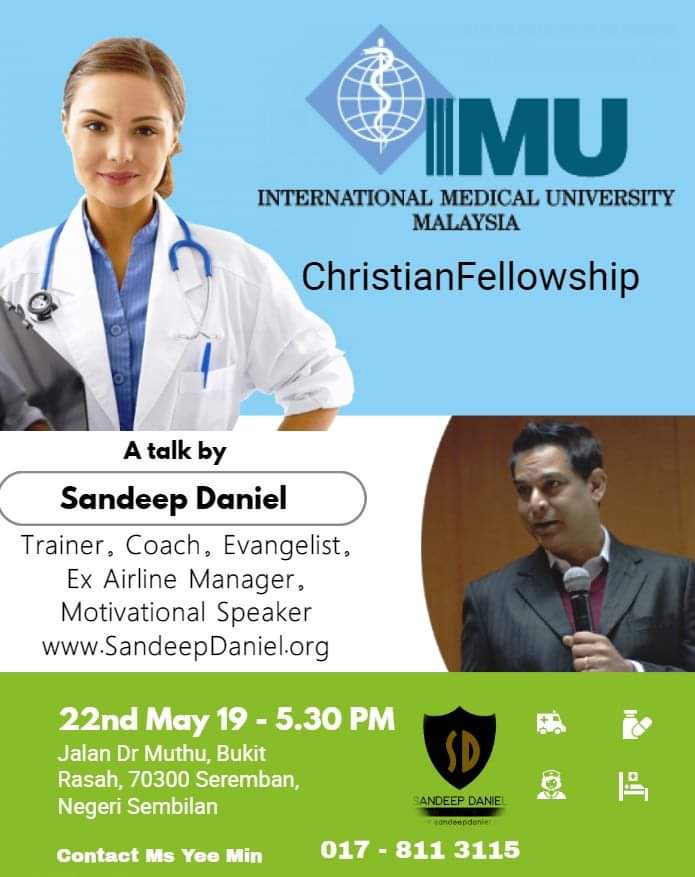This color-printed advertisement is a portrait-oriented flyer for a Christian Fellowship event hosted by the International Medical University (IMU) in Malaysia. At the top left, there's a photograph of a young female doctor with brown hair, wearing a white lab coat and a blue stethoscope around her neck, her right hand propped on her hip and holding a green cuff. To her right is the IMU logo: a blue diamond shape containing a white globe and the medical snake symbol, followed by 'IMU International Medical University Malaysia' and 'Christian Fellowship' in black text. Below this, the flyer announces a talk by Sandeep Daniel, who is described as a trainer, coach, evangelist, ex-airline manager, and motivational speaker, with a link to his website www.sandeepdaniel.org. A section toward the lower part of the flyer features Sandeep Daniel's photograph on the right, resembling him making a speech. At the bottom, a green horizontal border lists the event date, May 22, 2019, at 5:30 PM, and provides detailed location information: Jalan Dr. Muthu, Bukit Rasa, 70300 Seremban, as well as a contact number, 017-811-3115, for further inquiries.